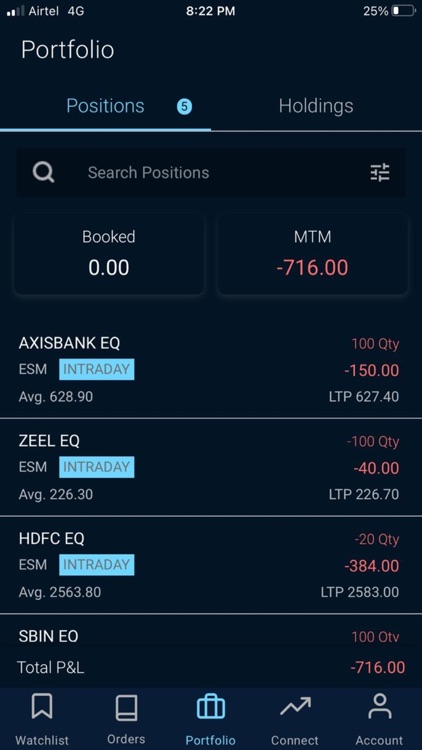Screenshot of a mobile investment portfolio on a smartphone with a black top border displaying network details and battery status. The top bar shows an Airtel 4G connection, time as 8:22 p.m., and a battery level at 25%. 

Below this, two main tabs are labeled "Portfolio" and "Holdings". The "Positions" tab under "Portfolio" is currently selected. A search box for "Search Positions" is present, and beneath it are sections for "Booked" showing 0.00, and "MGM" indicating a negative 716.00.

The portfolio lists various equity holdings: Axis Bank EQ, Zeal EQ, HDFC EQ, and SBINEO. The total profit and loss (P&L) at the bottom show a deficit of 16.00.

At the very bottom of the screen, navigation tabs are visible for Watchlist, Orders, Portfolio (currently highlighted), Connect, and Account.